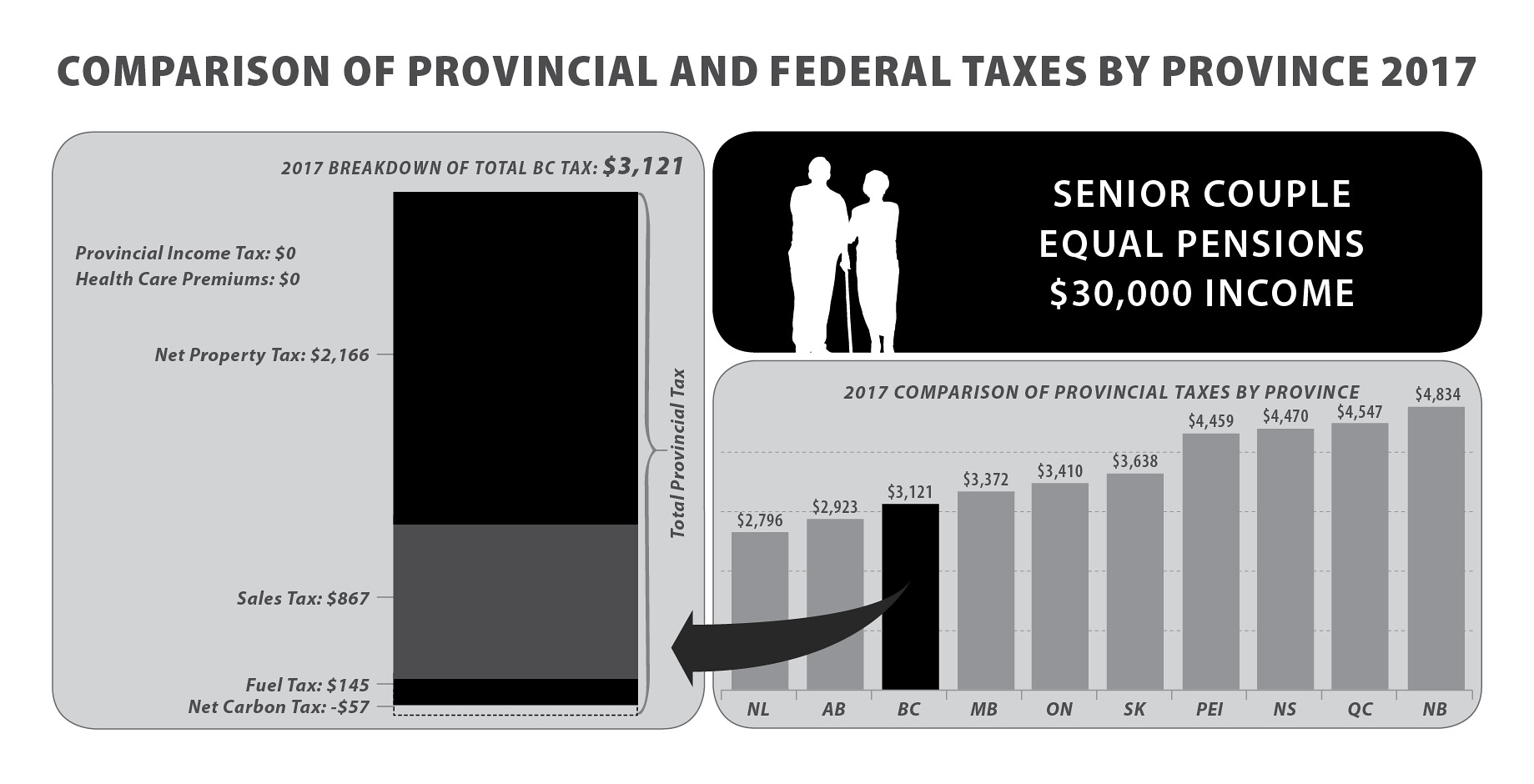The image is a black, white, and gray chart titled "Comparison of Provincial and Federal Taxes by Province 2017." It includes three sections. On the left is a detailed breakdown of the total BC tax amounting to $3,121, divided into categories: Net Property Tax ($2,165), Sales Tax ($867), Fuel Tax ($145), and Net Carbon Tax ($557). In the middle section, there is a depiction of a senior couple, labeled as having equal pensions with a combined income of $30,000. Adjacent to this, on the right, is a vertical bar graph comparing these taxes across different provinces, emphasizing the detailed breakdown for British Columbia from the first section.